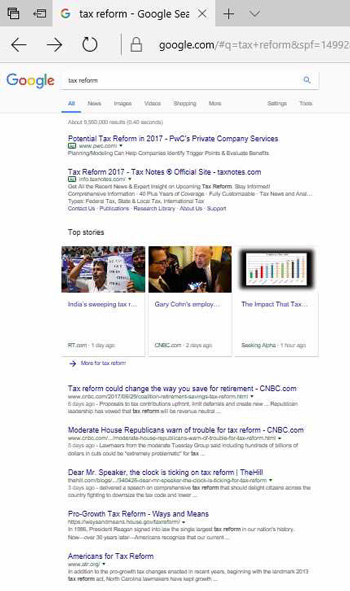The image portrays a screenshot of a Google search results page on a website with dimensions approximately two and a half to three times taller than it is wide. At the top, we see an open browser tab displaying the Google icon, with the title "tax reform - Google Search" followed by a black X indicating the option to close the tab. The tab is set against a medium gray background that transitions to a lighter gray in the next section which encapsulates the typical browser navigation bar.

In this navigation bar, familiar icons are present including the left and right arrows for navigation, a refresh button, and the secure connection padlock icon, followed by the Google site URL. Below this, the interface shifts to Google's homepage layout, featuring the multicolored Google logo on the left and a search bar to its right. The search term "tax reform" is already entered in the search bar with a magnifying glass icon (search button) to the far right.

Directly beneath the search bar, a menu allows users to filter results by categories like All, News, Images, Videos, Shopping, More, Settings, and Tools. The 'All' category is currently selected, highlighted in blue and underlined.

The search results that follow show typical text links under titles in a purple-blue hue, though some text appears blurry and hard to read. Example titles visible include "Tax Reform in 2017," "PwC's Private Company Services," and "Tax Reform 2017 Tax Notes," along with the URL "official site-taxnotes.com."

The overall format is indicative of a standard Google search results page, providing a familiar interface.